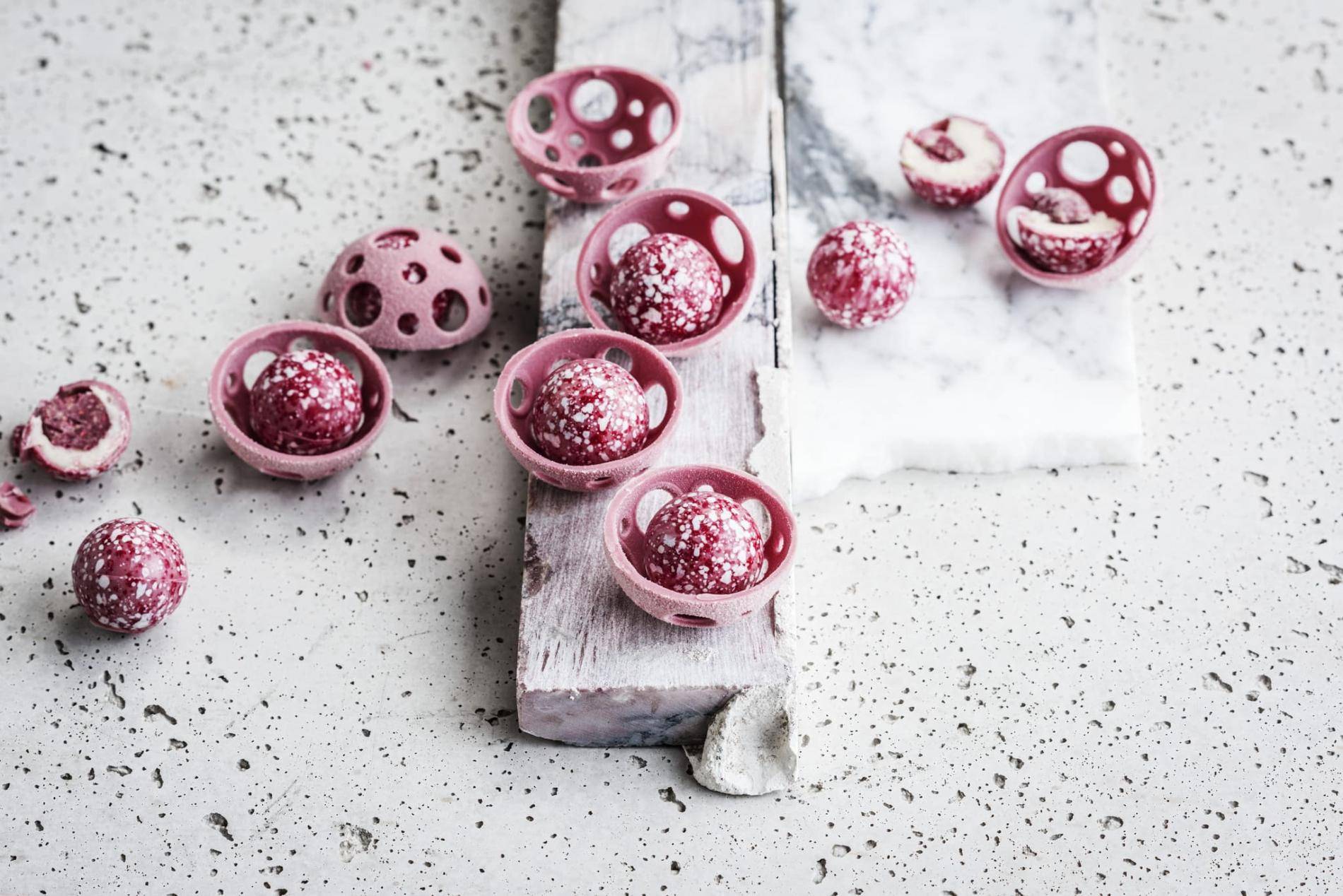The image depicts a collection of hollow, pink plastic spheres resembling half-circle casings dotted with Swiss cheese-like holes. These casings house perfectly round, speckled balls that are primarily white with red flecks. Some of these spherical casings are broken open, revealing the layered contents within. Each ball has a white exterior layer and a red core inside, though it is unclear whether these are fruit, food items, or another type of object. The scene is set against a flat, porous white surface that resembles stone with visible air bubble imperfections, suggesting it was molded. Additionally, some of these white and red speckled balls are resting on what appears to be a piece of white-painted wood.